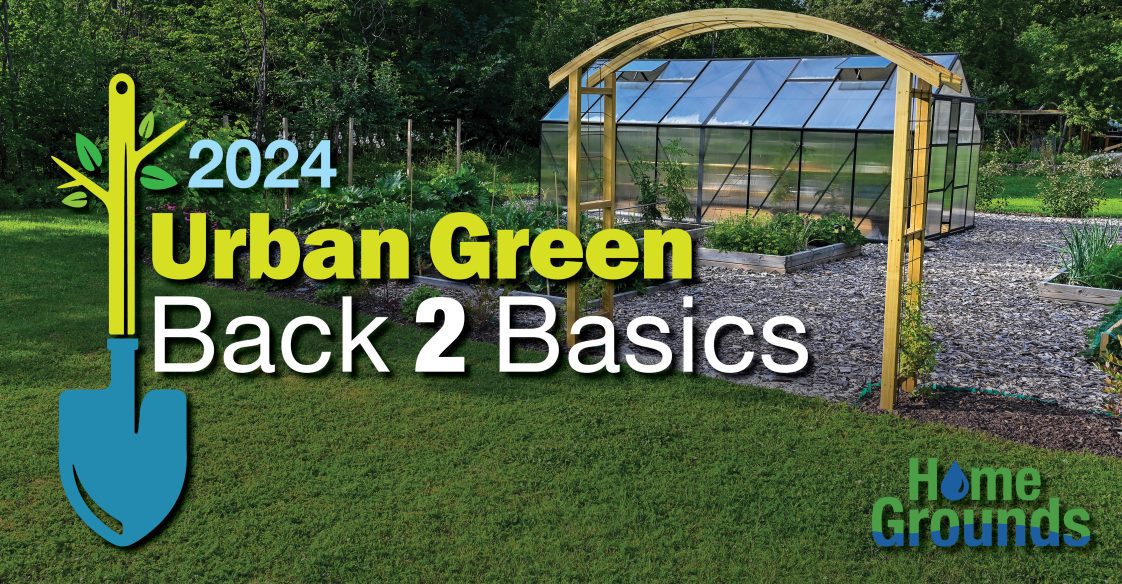The image is an advertisement depicting a picturesque garden scene with a focus on a greenhouse. The foreground features a lush, soft green lawn leading up to the garden area. At the entrance to this space, a wooden pergola with an arched roof stands prominently. Inside the garden, the space is adorned with several raised garden beds and planter boxes filled with various plants. The ground inside is covered with rocks. The greenhouse, positioned towards the right, is constructed of metal and glass. In the background, there are numerous trees, suggesting the edge of a forest.

The advertisement includes text prominently displayed at the center left, reading "2024 Urban Green Back to Basics." Additionally, there is a graphic of a blue shovel with a yellow handle growing branches and leaves, symbolizing growth and nature, situated towards the left side of the image. In the bottom right corner, a logo reads "Home Grounds," tying the scene to its advertiser.